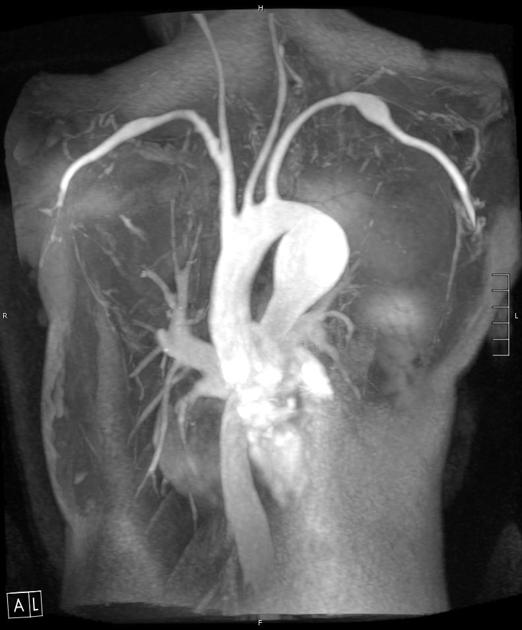This image appears to depict an x-ray of a human body viewed from the back. The x-ray, which is in black and white, displays the shoulders and the upper back with notable internal structures illuminated against a dark background. Central to the image is a distinctive large, white curved shape, reminiscent of a goose head bent over and flat on one side. This central shape is flanked by two prominent, bright white lines that curve outward and upward, possibly indicative of bones or significant anatomical features extending over the shoulders.

Additionally, there are faint lines extending upwards towards the neck area. In contrast to these bright elements, sections of the body exhibit varying shades of gray, possibly representing softer tissues or different internal organs. The left side of the image hints at visible ribs, whereas the right side appears less distinct.

A noteworthy element is a cube in the lower left corner labeled with the letters 'A' and 'L' on its faces, which may serve as a reference or marker. Meanwhile, towards the right side of the image, there’s a faint indication of horizontal lines that might represent a chart or additional markings. Overall, this detailed x-ray encapsulates a complex view of the upper human body, displaying intricate internal details with a mix of bright and shaded areas.